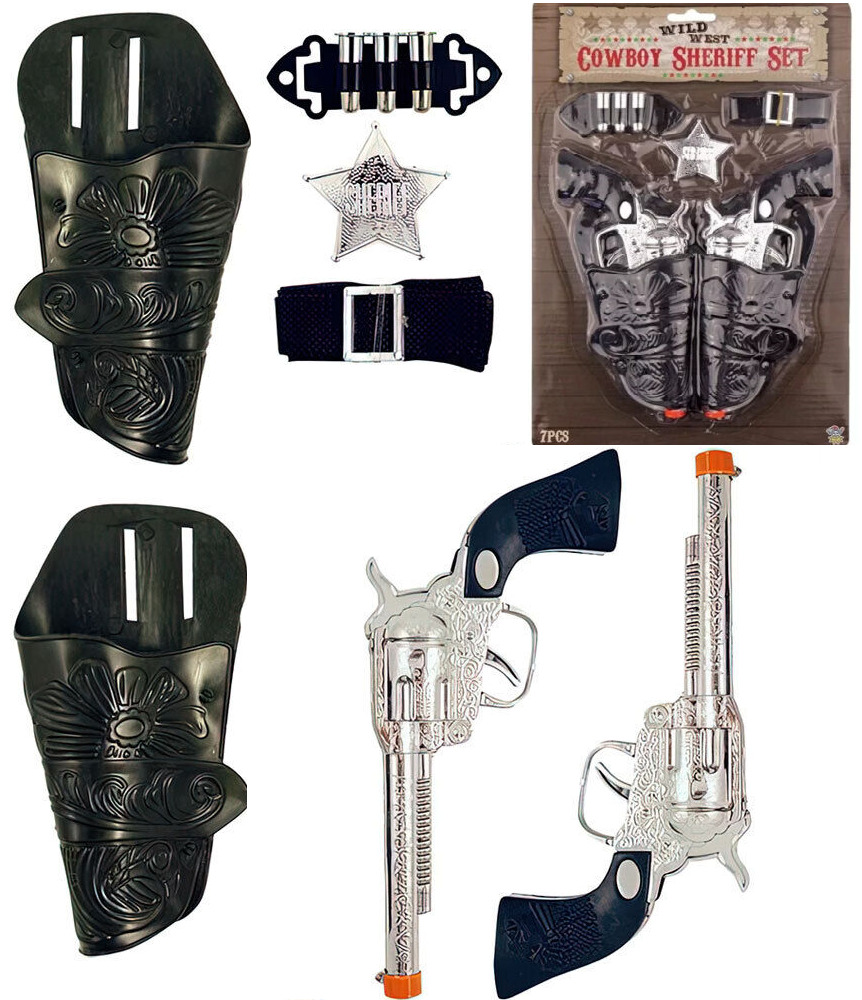The image showcases a comprehensive Wild West Cowboy Sheriff toy set. The set includes two silver pistols with distinctive blue handles and safety orange caps to indicate they are toys. The set also features two black plastic holsters adorned with floral designs, designed for both the right and left sides, which can be attached to the provided black belt. Additionally, there's a shiny silver sheriff's badge with the word "Sheriff" prominently displayed. The set includes a black belt attachment that securely holds three silver toy bullets. The individual elements of the set are displayed neatly alongside a packaged image that depicts the entire set assembled, emphasizing its role-playing potential for aspiring young sheriffs.